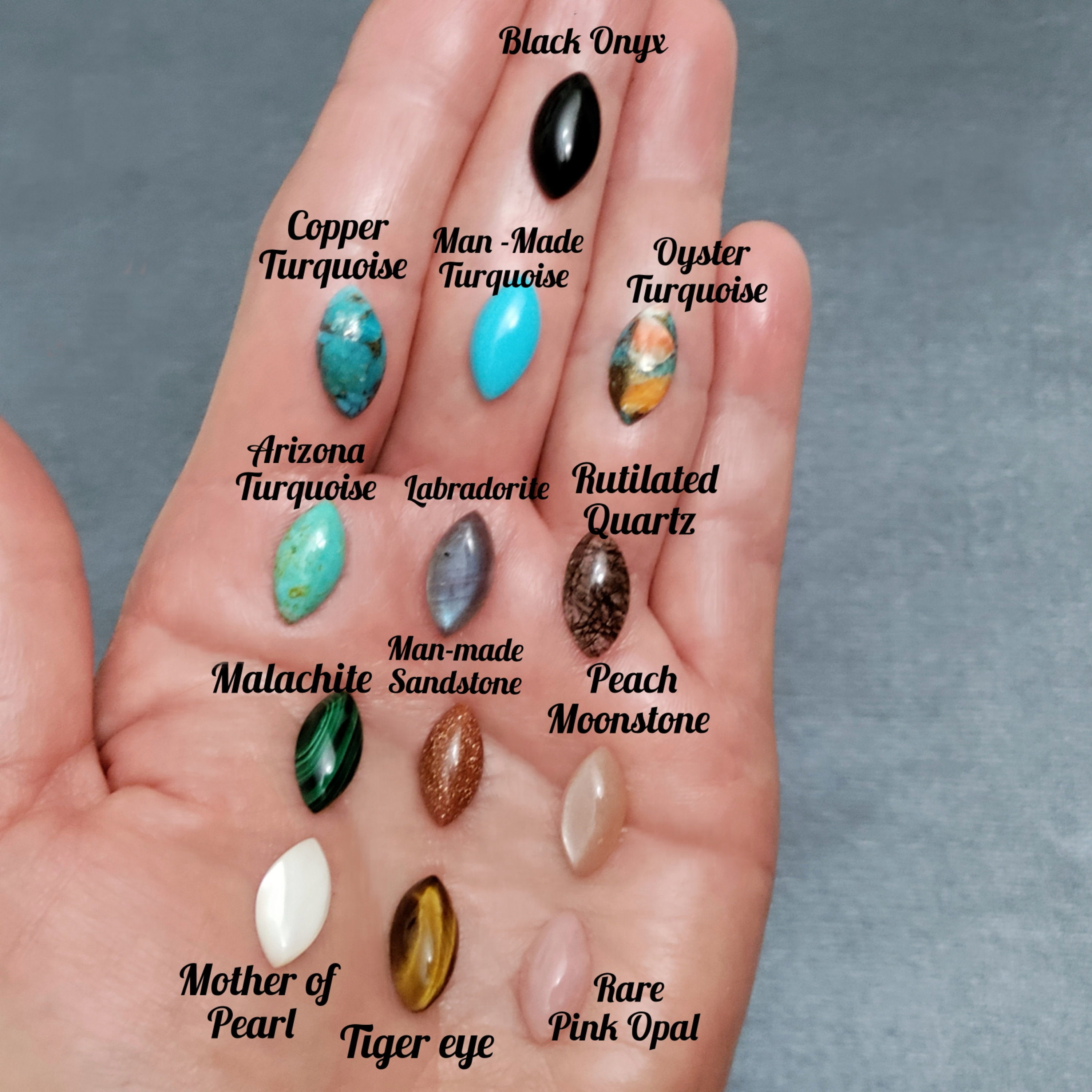The image features a close-up of an open hand against a gray background, holding and displaying thirteen oval-shaped semi-precious stones of various colors and origins. Each stone is labeled in black italicized text, and the names are clear and easy to read. The stones, arranged in a detailed layout from the wrist to the fingertips, include: at the bottom, from left to right, Mother of Pearl, Tiger Eye, and Rare Pink Opal; above those, Malachite, Man-Made Sandstone, and Peach Moonstone; further up, Arizona Turquoise, Labradorite, and Rutilated Quartz; and towards the top, Copper Turquoise, Man-Made Turquoise, Oyster Turquoise, and finally at the tip of the middle finger, Black Onyx. The stones, approximately the size of a small bead, exhibit a diverse palette ranging from vibrant blues and greens to soft pinks and rich blacks, each meticulously captured to show its unique characteristics.